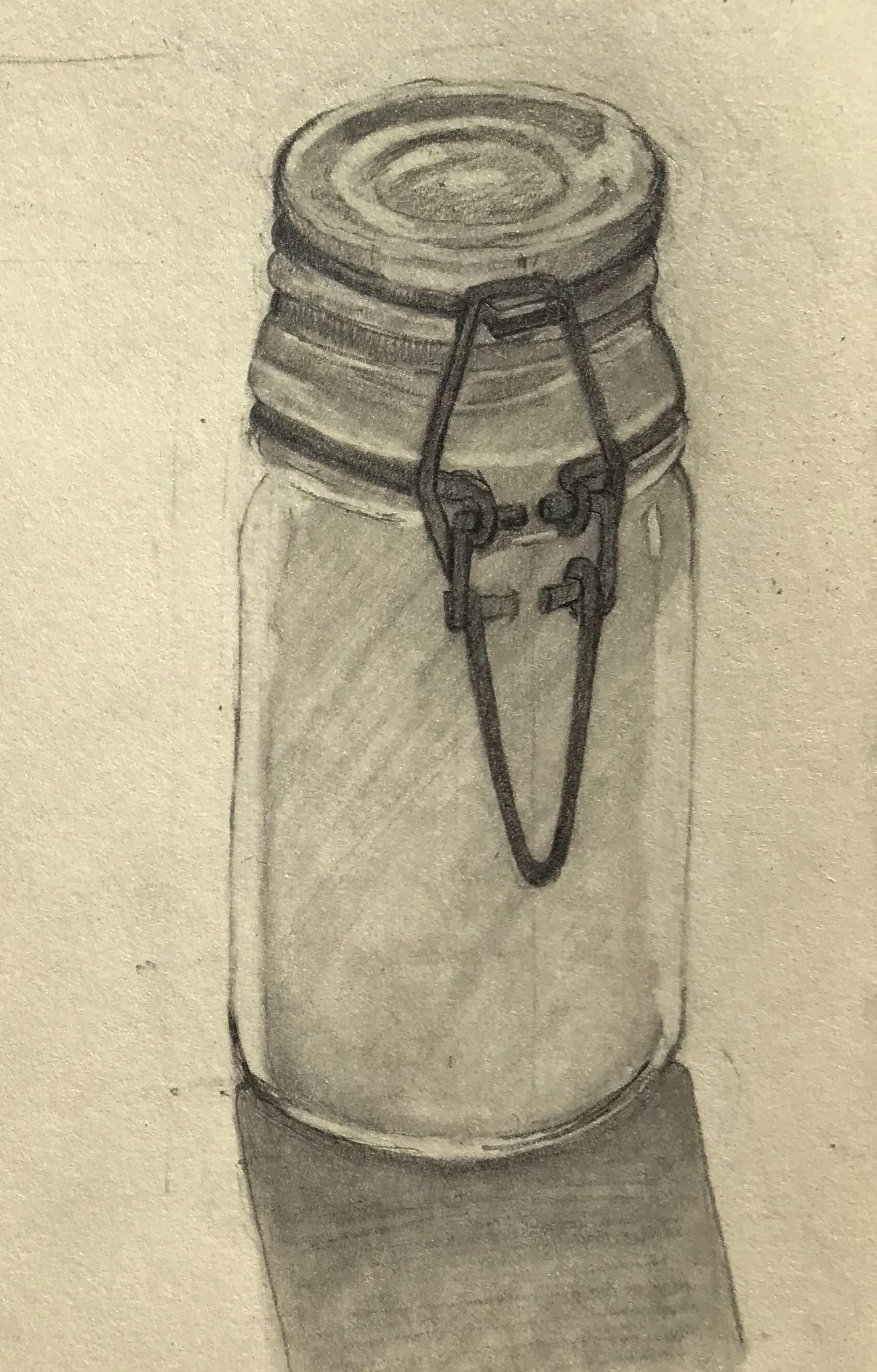The artwork is a detailed pencil sketch of a mason jar prominently displayed on a white to cream-colored paper. The jar features a twist-off lid with a hinge mechanism, illustrated from the back view, where the hinge is clearly visible. The drawing uses grayscale shading extensively to emphasize the intricate details of the jar, such as the rigid neck, the indented lid, and the dark, silver-colored clasp that secures the lid in place. The lower part of the jar is shaded very dark, casting a distinct shadow towards the bottom of the page, enhancing the three-dimensional effect. The overall background is lightly grayed, adding subtle texture and creating a glow effect that suggests the jar is in a dimly lit room. The pencil work varies in intensity, with lighter strokes creating softer areas and darker strokes highlighting more pronounced features, giving the jar a realistic and textured appearance. The jar appears to be empty, with no contents visible inside.